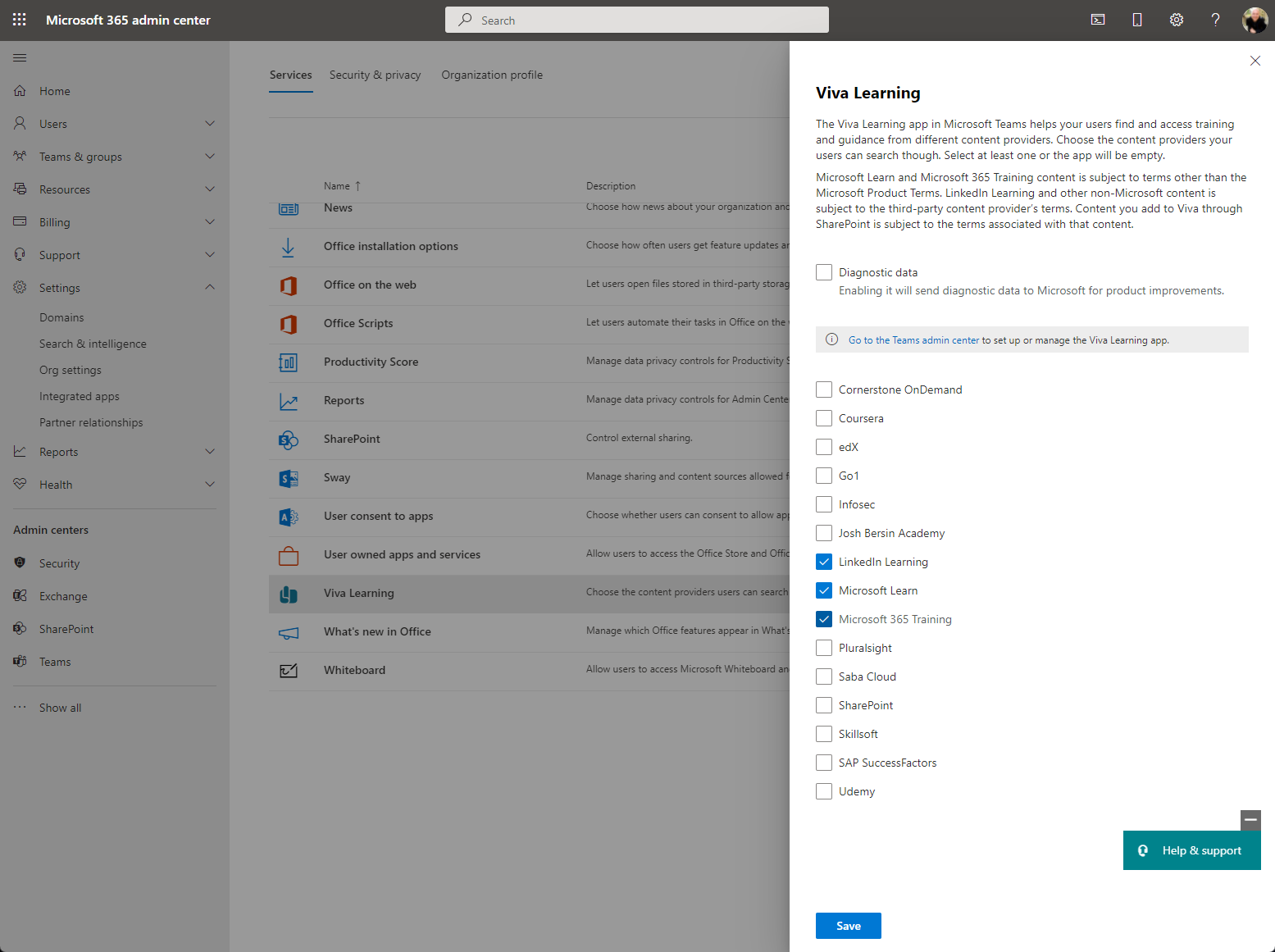This screenshot displays the Microsoft 365 Admin Center, evident from the website's interface shown in the image. The top left corner of the page distinctly labels it as the Microsoft 365 Admin Center. The page features a black and light gray banner across the top. 

On the right-hand side, there is a user profile icon situated at the top, suggesting an administrative account or user profile is logged in. The image also includes a sidebar on the right, which appears to be an overlay that has been activated by clicking on an option within the main interface. The title of this sidebar is "Viva Learning," indicating that it is a section dedicated to this specific feature of Microsoft 365.

Below the "Viva Learning" title, there is a brief description that is somewhat difficult to decipher in the screenshot, presumably explaining the features or benefits of Viva Learning. At the very bottom of the sidebar, there are several checkboxes corresponding to various resource options. These options are listed vertically and include:

- Commercials on Demand
- Courses
- edX
- Go1
- InfoSec
- Josh Berin Academy
- LinkedIn Learning
- Microsoft Teams
- Microsoft 365 Training

Out of these options, the boxes next to LinkedIn Learning, Microsoft Teams, and Microsoft 365 Training are checked, indicating selected preferences or enabled resources within the Viva Learning module.